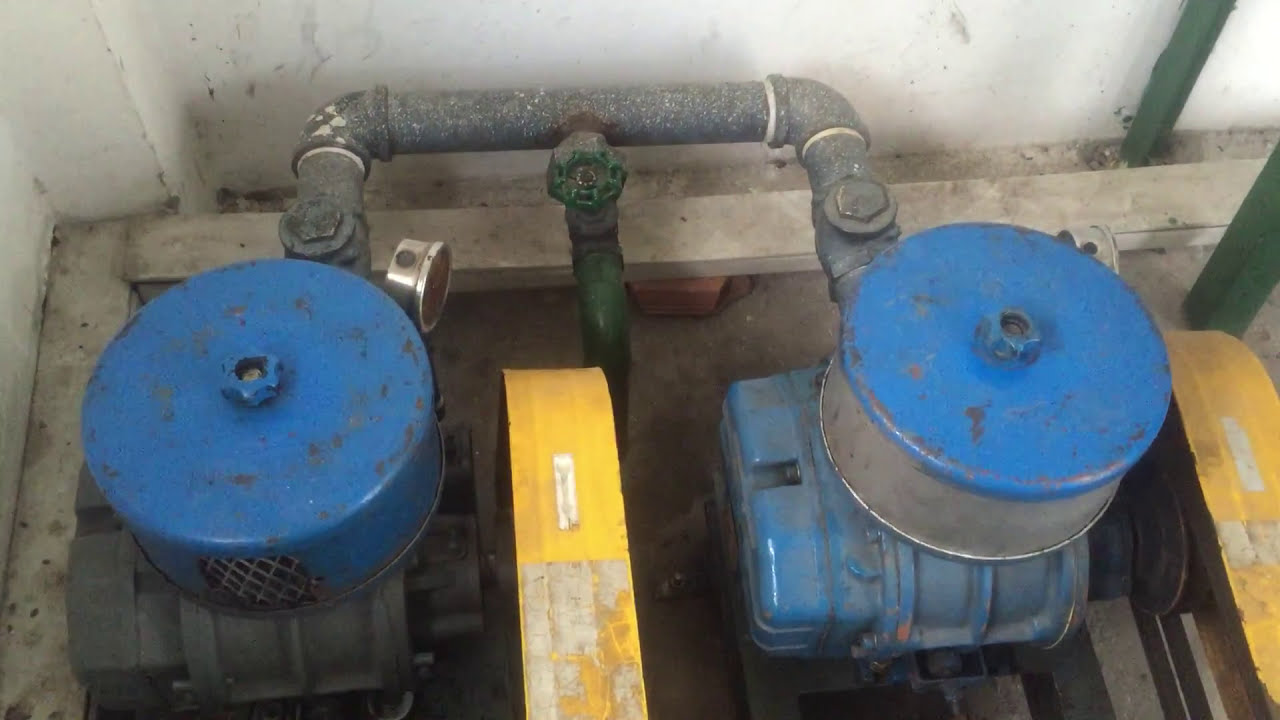The image showcases a complex plumbing setup or an engine system installed against a dirty, soiled concrete wall in a dingy corner area. The primary components include two blue, circular metal drums, which are likely part of an engine or pump system. These drums are interconnected by a large gray pipe, with an additional green pipe extending downward from the middle of this gray pipe. In between and on either side of the blue drums, there are yellow metal sections resembling turnbelts or pulleys, which are covered by shields for protection. These yellow sections bend downwards and then run up and across, creating a symmetrical layout.

The setup also features an array of smaller parts: visible are blue covers, likely for filters, and other metal pieces that might be small motors. These parts are integrated via various pipes and valves, including water piping, a valve, and an analog gauge. The entire assembly appears to be embedded into the wall, with a cement backdrop showing signs of age and grime. The presence of a filter with a mesh screen on the left and a simpler plastic-covered filter on the right further accentuates the system's intricate design and utilitarian purpose.